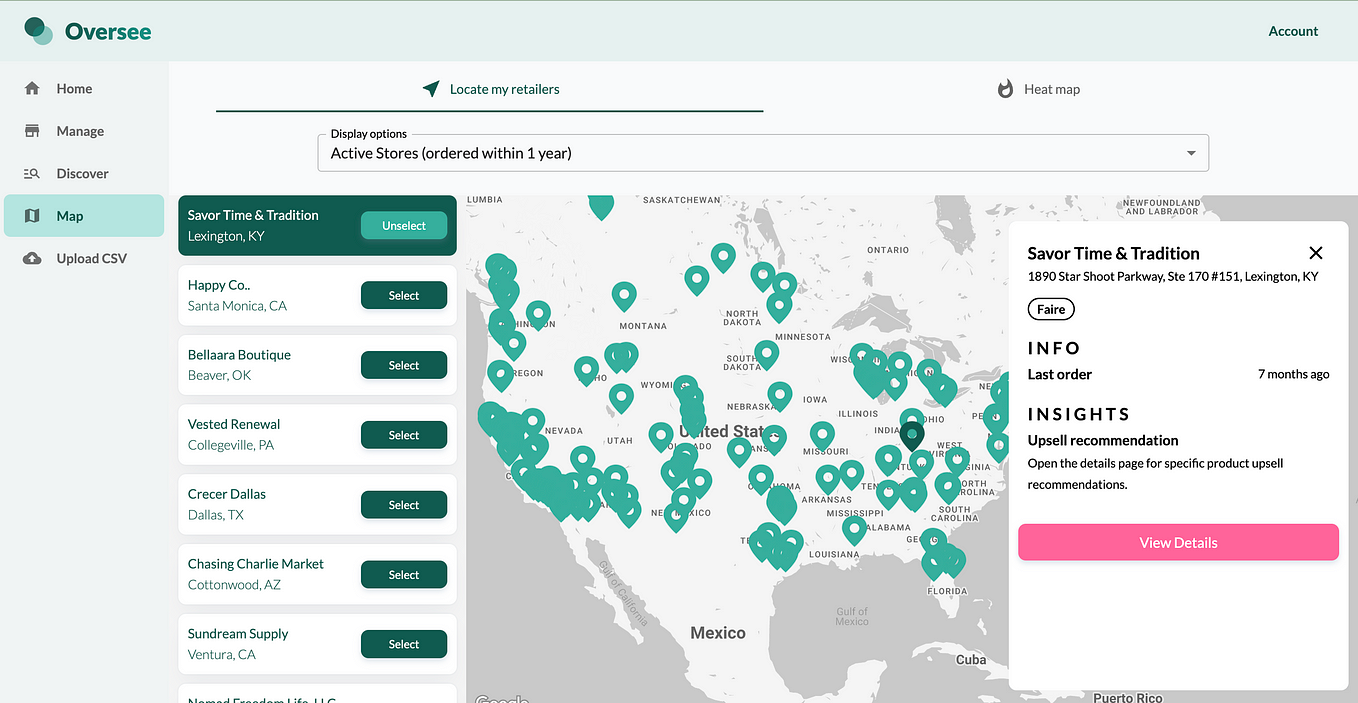The image is a horizontally rectangular screen grab from a software application, with the lower portion cropped out. The top left corner features the label "Oversee" in green, and on the top right, "Account." Beneath "Oversee," a vertical menu lists options: Home, Manage, Discover, Map, and Upload CSV. The "Map" option is highlighted, causing the right side of the screen to display a map of North America. The map is densely populated with green markers, mainly concentrated in the United States, with a few extending into Canada.

On the right side, a pop-up window partially obscures the northeastern U.S. This window contains detailed information under the heading "Savor Time and Tradition, 1890 Starshoot Parkway, Suite 170, Number 151, Lexington, Kentucky." Below, it provides operational insights such as "Last Order: Seven Months Ago," along with a section titled "Insights" featuring an "Upsell Recommendation" prompt. This encourages users to "open the details page for specific product upsell recommendations." A prominent pink button labeled "View Details" in white text invites further action.